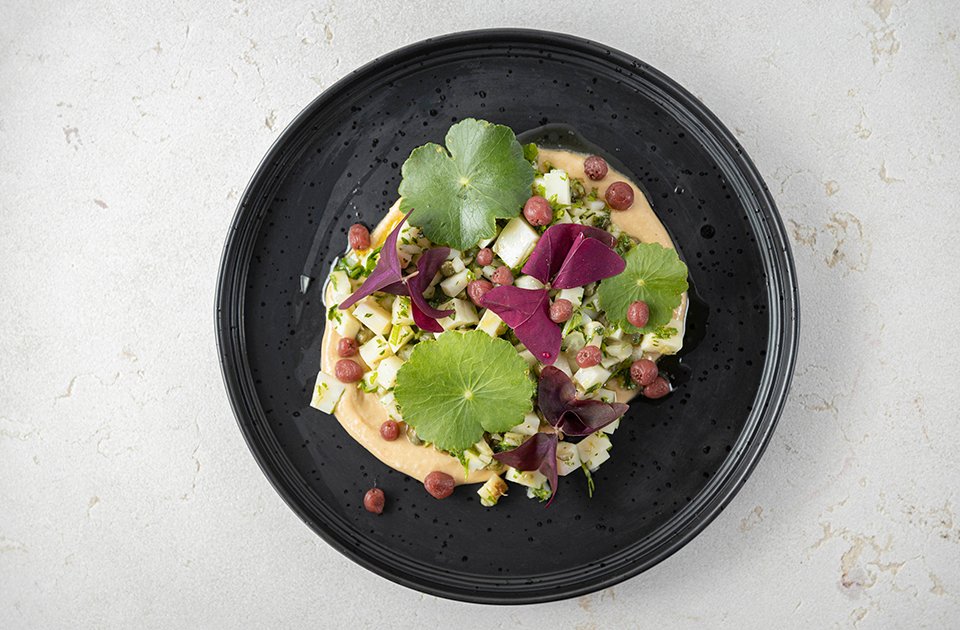The image showcases an overhead aerial view of a black plate centered on a white, textured stone table. The plate features a visually appealing and sophisticated dish that conveys a high-end culinary presentation. The food comprises a pale peach-colored sauce or puree at its base. Atop the sauce sits an assortment of ingredients: various-sized cubes of white cheese, small purple berries, and garnishes that include both green and purple leaves. The green leaves are notable for their circular shape and serrated edges. Additionally, there are purple shavings that could be from flowers or beets, adding a pop of color to the arrangement. The plate also appears to have drops of water on its surface, suggesting that it is slightly wet. This indoor setting emphasizes the artistry and complexity typical of fine dining cuisine.